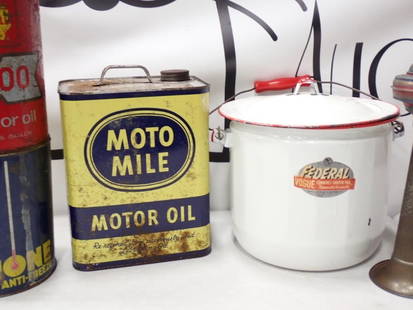The image showcases an intriguing collection of old, weathered items displayed on a white countertop. Dominating the scene is a vintage yellow Motomow motor oil can, prominently featuring a blue label with the brand name "Motomow" in yellow and "motor oil" written within a blue bar at the bottom. The can, designed with a silver handle and screw cap, likely holds around a gallon of oil. Flanking this central oil can is a white chamber pot with the logo "Federal" inscribed on its side. This pot is detailed with a red trim around its lid and a red handle attached to a wire, giving it a distinct appearance. To the left of the Motomow can, two smaller, dirty cans are stacked. The bottom one is blue with yellow writing, likely indicating "ONE ANTIFREEZE," while the can on top is red with partial text "OR OIL," suggesting it too is an oil canister. The background features a white banner with dark blue or black writing, though the exact inscription is unclear. The overall ensemble presents an intriguing glimpse into a bygone era of automotive care.